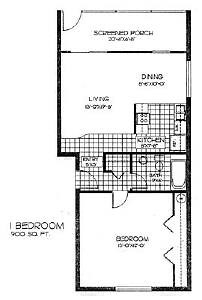This detailed drawing illustrates a floor plan for a 900 square foot house. The text is rendered in black, though some portions appear blurry. The floor plan features multiple labeled rooms. At the forefront, there is a clearly marked "Screened Porch," depicted as a rectangular shape. Below this area lies a square-shaped section labeled as "Dining Room," "Living Room," and "Kitchen," complete with detailed illustrations of kitchen appliances including a stove, refrigerator, and a kitchen door. Adjacent to this, another square denotes a "Bedroom," which includes a door for entry. Nearby, there is a room marked "Bath," containing a drawing of a bathtub. Additionally, to the left side of the plan, another "Bedroom" is specified, contributing to the cozy layout of this compact yet well-designed 900 square foot home.